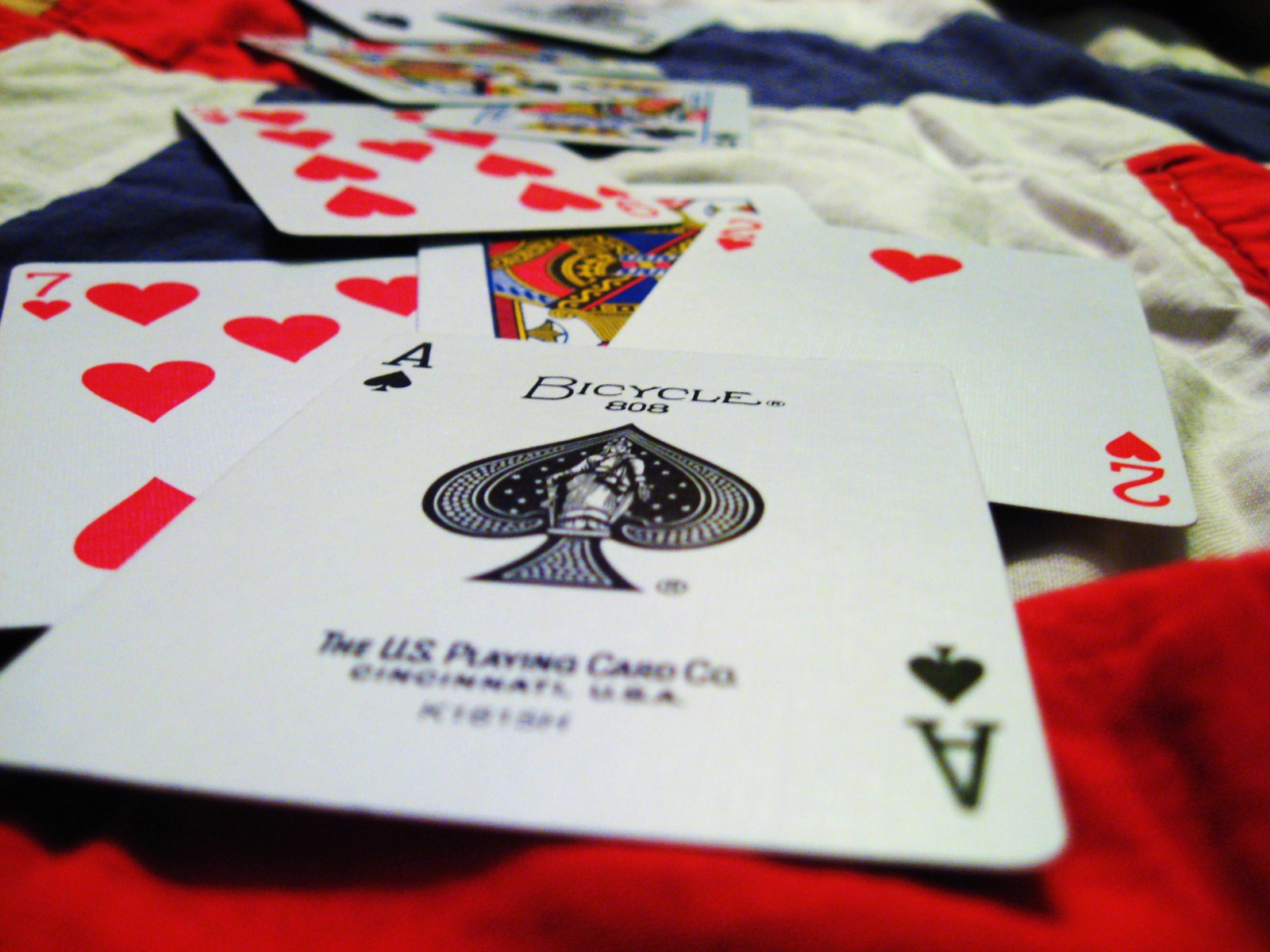This vibrant color photograph features a scattered arrangement of playing cards laid out on a red, white, and blue striped blanket, resembling a handcrafted quilt. At the forefront of the image is an Ace of Spades, prominently displaying the words "Bicycle," "808," and "U.S. Playing Card Company," indicating its origin from Cincinnati, USA. Surrounding the Ace are a variety of cards, including a 7 of Hearts, a 2 of Hearts, and a 9 of Hearts. Among the higher-value cards, a Queen is clearly visible, while another is partially obscured beneath the 9 and 2 of Hearts, likely a King. The cards are haphazardly strewn without any particular order, creating a casual and spontaneous display. The texture and colorful stripes of the quilted blanket add a cozy and nostalgic background to the scene, making the scattered playing cards the focal point of this detailed and captivating image.